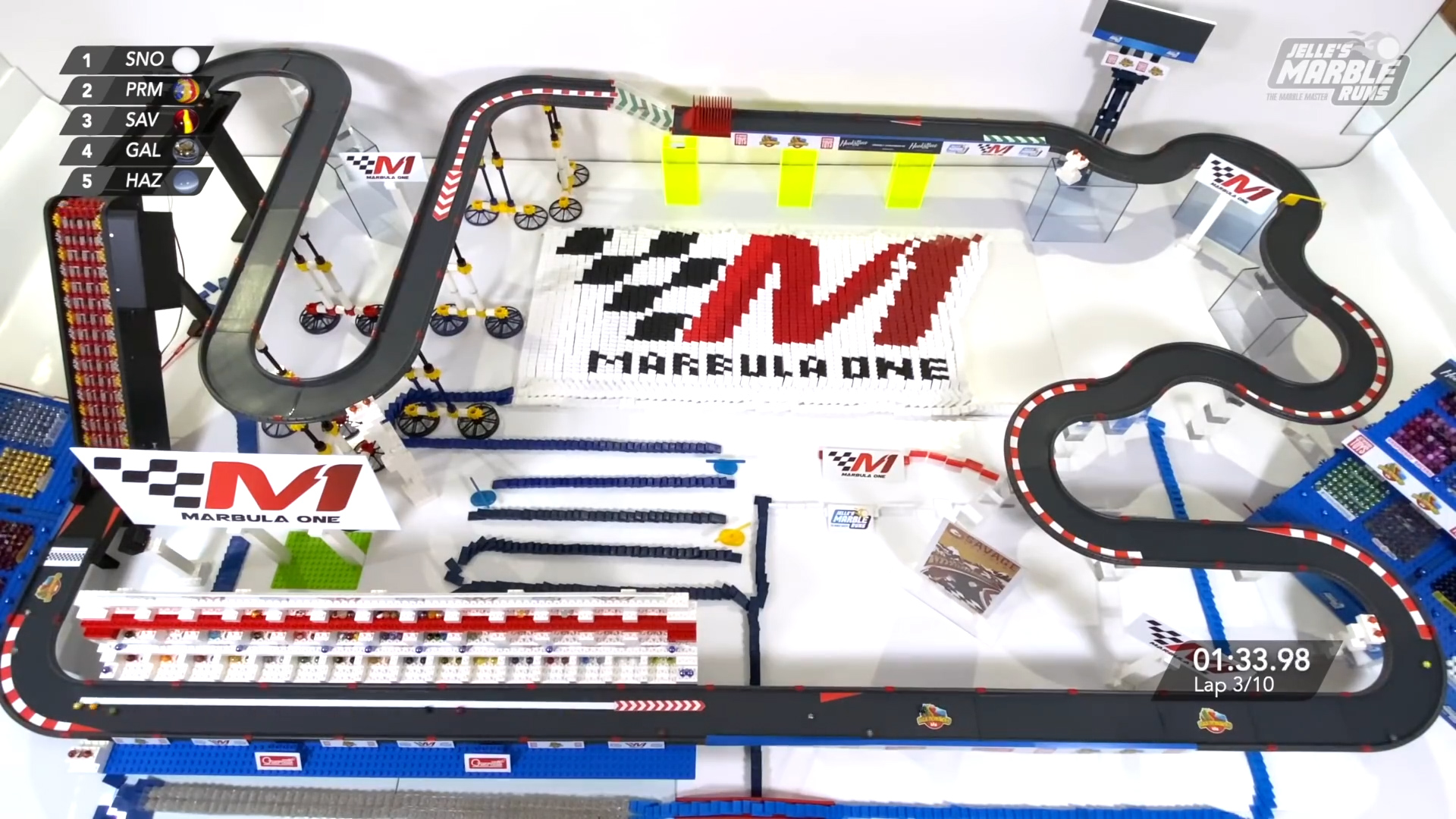The image depicts an intricate gaming device designed to simulate a racing track. The track features a continuous black roadway accented with sharp red and white stripes that add a sense of speed and urgency. At the center of the scene is a prominent black stand supporting a large, billboard-like screen. This screen displays a striking white sign. 

The background of the display is white and prominently features a large red "M" alongside black and white boxes. The text "MARBULA 1" is emblazoned across the sign in bold black lettering. Additional visual details include strips of navy and black that adorn the screen. 

To the left, there is a box marked with a big "M" that reads "Marlboro 1, Marbula 1." Below the billboard, along the outside of the track, lies a long white panel edged with a red stripe. The upper left corner of the image lists rankings in small black boxes: 
1. "SNO"
2. "PRM"
3. "SAV"
4. "GAL"
5. "HAZ."

Adjacent to this list is a vertically oriented black box featuring streaks of red and brown, while a blue box appears to its left. On the far right side of the image, the text "Jellies Marble Rules" is clearly displayed. The bottom right corner shows the sequence "01-33-98-3-10," potentially indicating game timings or scores. 

Overall, the scene captures the essence of a sophisticated racing game, combining vibrant graphics and detailed elements to create an immersive gaming experience.